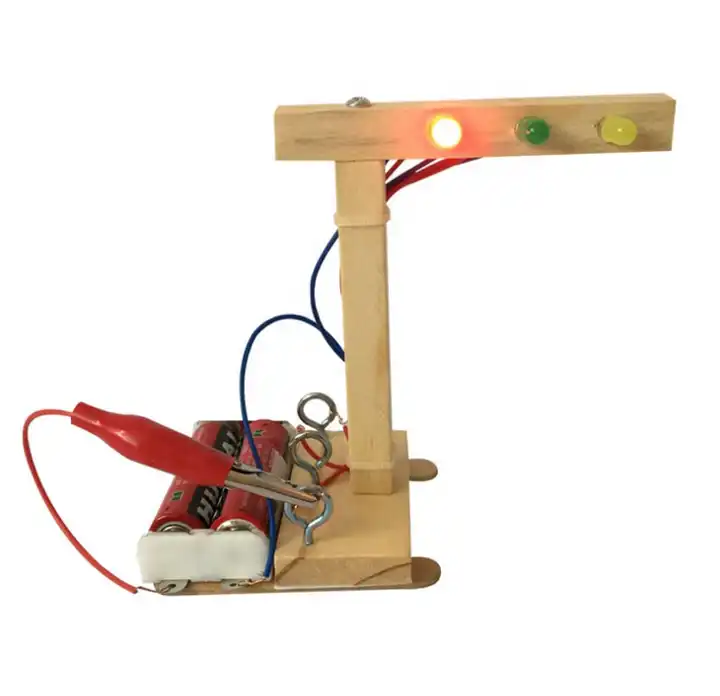This photograph depicts a small, possibly handmade, electrical contraption, similar to what one might find at a science fair or in a DIY tutorial. Set against a plain white background, the device features a wooden base with an unfinished wood structure forming an upside-down L shape. At the top of this structure, there are three lights: white, green, and yellow, with the white light on the left currently illuminated.

Near the base of the wooden structure, three metal rings (or screw-in eyes) are attached, each facilitating a different connection. A red-handled metal clamp (alligator clip) is affixed to one of these rings. Powering the contraption are two red batteries, connected by blue and red wires. The blue wire runs from the battery pack up to the light post, while the red wire with the alligator clip connects to the nearest screw-in eye. The layout includes an assortment of power wires in black, blue, and red, all contributing to this rudimentary lighting circuit.

Overall, this intricate assembly appears to be a part of an educational experiment, showcasing fundamental electrical concepts through its simple yet functional design.